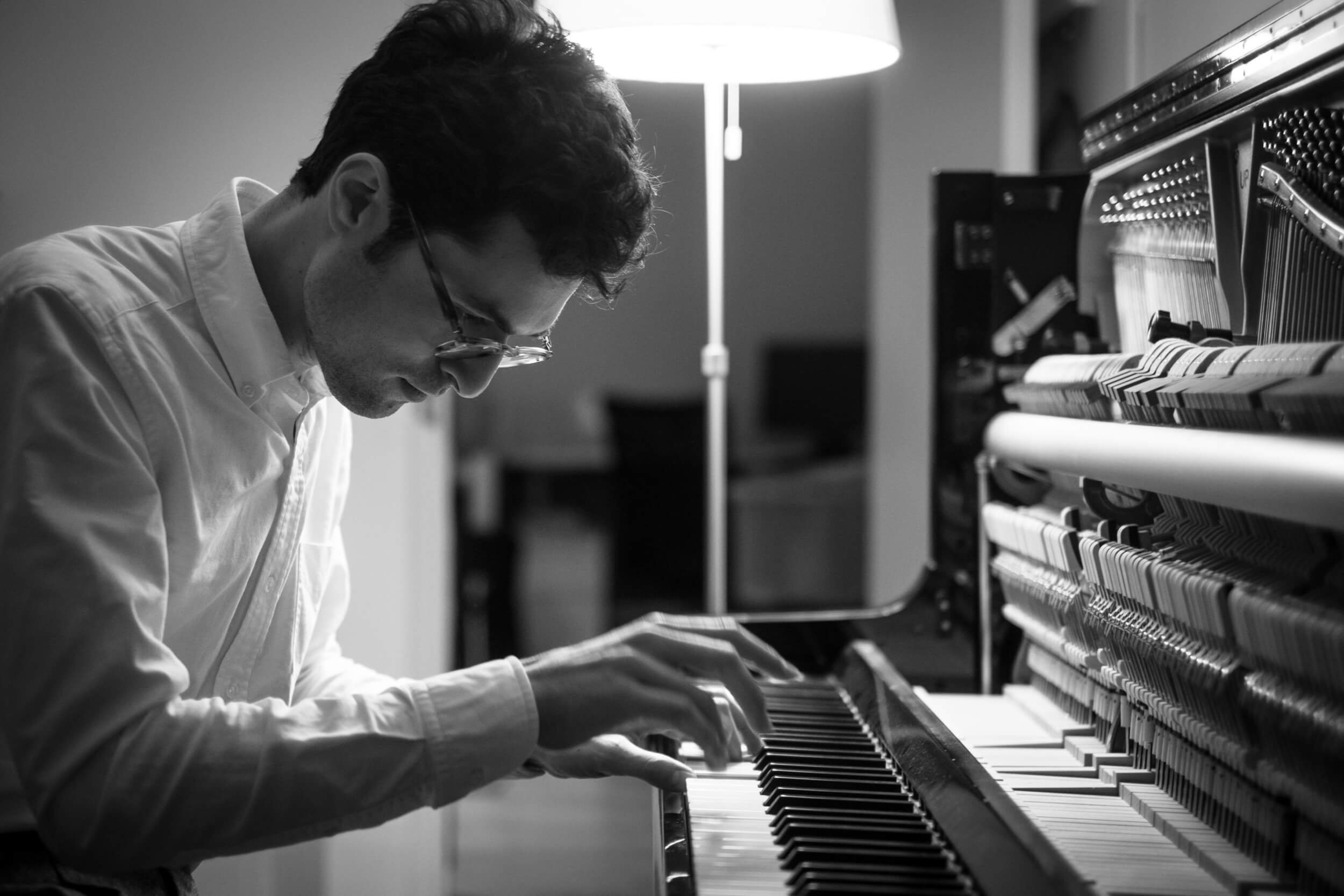In this black-and-white photograph, a man with dark hair and glasses is fully engrossed in playing a stand-up piano. He is wearing a white, collared, long-sleeved shirt and is intently focused on his hands, with his left hand pressing a chord on the keys and his right hand poised just above them. The image captures the moment with great clarity on the man and the piano, showing intricate details like the piano’s opened top, revealing its inner workings where the keys strike the strings to produce sound. The scene is set in what appears to be a house or a room, though the background is very out of focus. There is a tall lamp centrally positioned in the background, its thin rod and shade discernible, casting a glow over the scene. The background also hints at walls and an open doorway, contributing to the intimate and focused ambiance of the photograph.